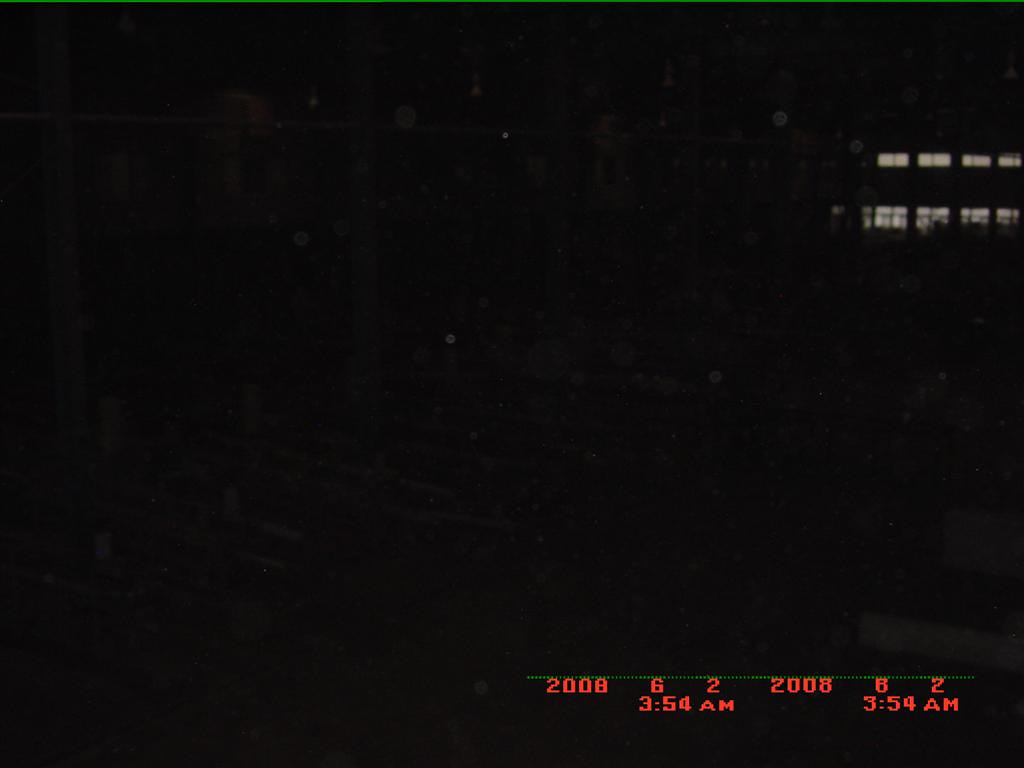This photograph, taken during nighttime, is predominantly dark, rendering most details almost invisible. However, in the top right corner, an illuminated apartment building is partially visible. The building has two stories, with the ground floor showing four sets of double windows, each brightly lit. The second floor mirrors this layout with four single windows also aglow. In the bottom right corner of the image, a timestamp is notable, showing "2008 6 2 2008 6 2" and "3:54 a.m." in bright red text, accompanied by a row of green dots above the date, suggesting the possibility of this being security camera footage.